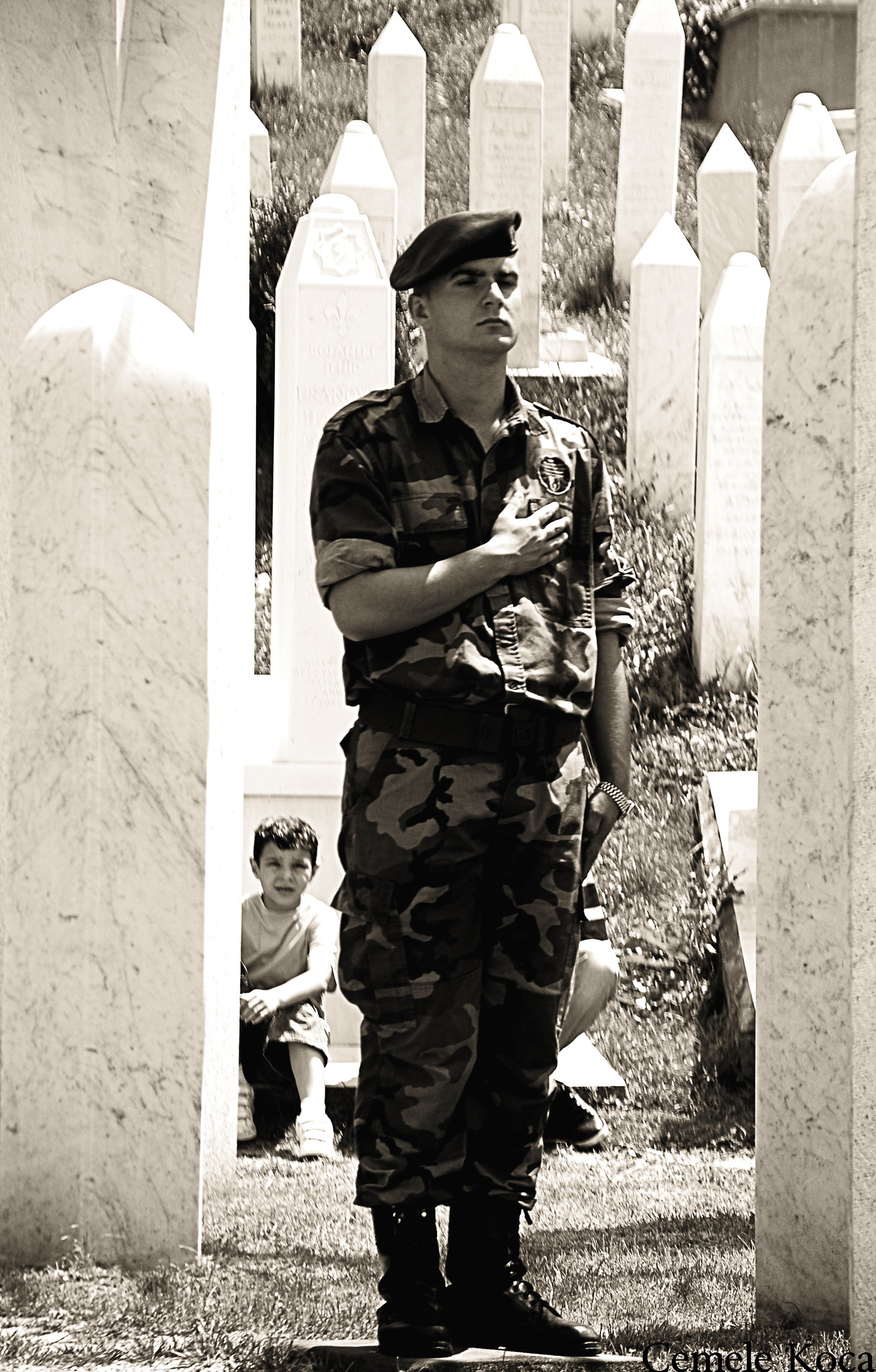This evocative black and white photograph captures a poignant scene set outdoors during the daytime. Central to the image is a somber soldier standing at attention, with his right hand over his heart. He is dressed in full camouflage fatigues, including a camouflaged shirt and pants, complemented by black combat boots and a dark beret on his head. His gaze is directed off into the distance, adding to the contemplative mood of the scene.

Behind the soldier, a young boy can be seen sitting on the ground. The boy is dressed in short pants and a light-colored t-shirt, providing a lighter contrast to the solemnity of the soldier’s attire. The setting appears to be a cemetery, as suggested by the numerous tall, white marble obelisks and pillars that surround them. The soldier's stance and the cemetery setting hint at an act of honoring fallen comrades. A grassy area extends behind him, leading up to a small hill adorned with more marble columns, reinforcing the solemn atmosphere of remembrance that pervades the image.